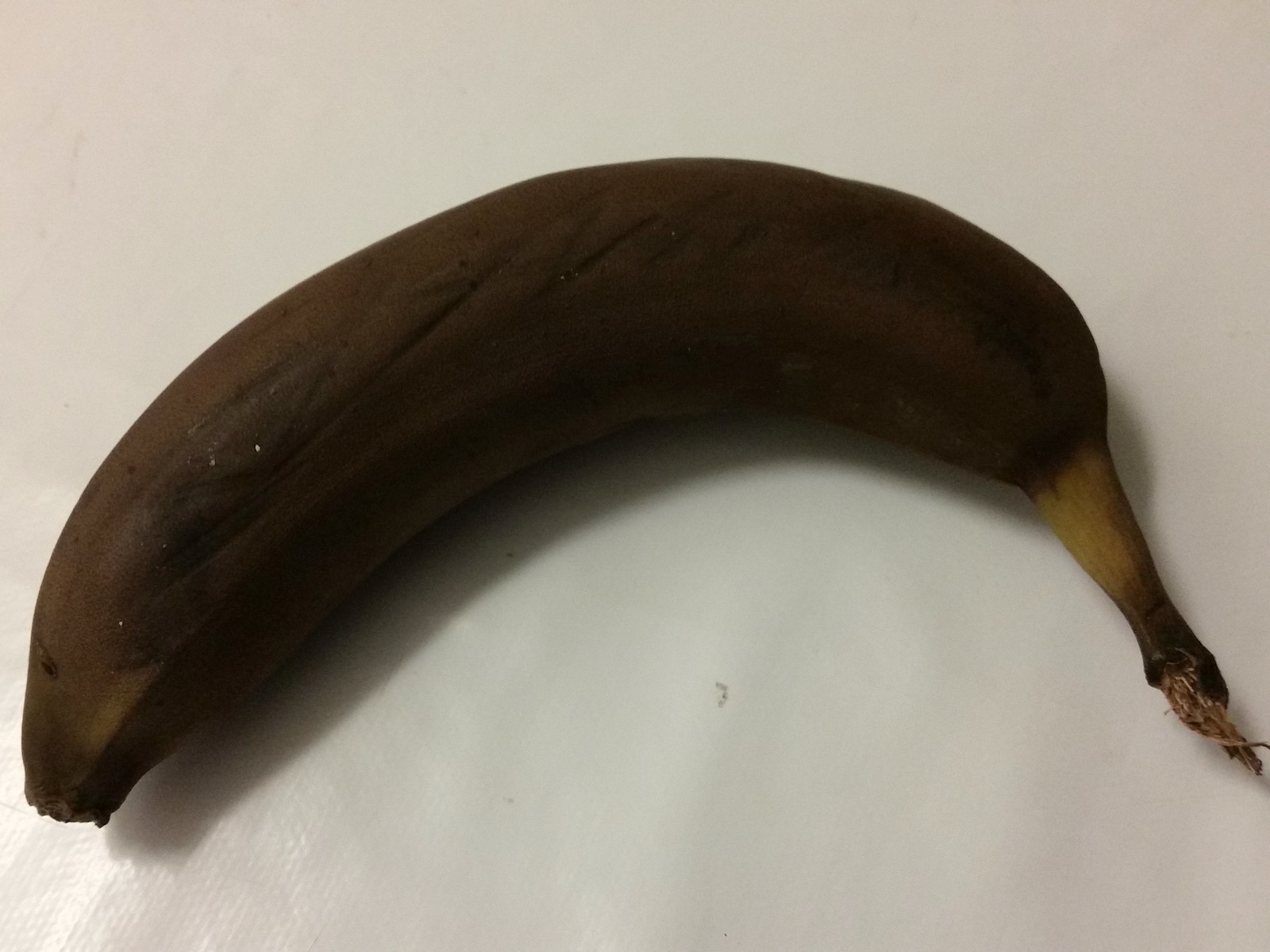The photograph captures an overripe banana, lying on an off-white, uneven surface that could be a tablecloth or countertop. The banana, arcing like a rainbow, has its stalk pointing downwards at a four o'clock position, while its tip points into the bottom left corner. The banana's skin is predominantly dark brown with black spots, suggesting significant overripeness. A small yellow patch is visible near the neck of the stalk, transitioning back to a dark color. Fine, dark-brown fibers dangle from where the banana was detached from the branch. There is a distinct highlight just beneath the tip of the banana on the left side, indicating an artificial light source from above the left, creating a shadow along the inside curve toward the bottom of the image. The surface of the banana has striations and indentations, adding texture that suggests it may have been pressed against another object.